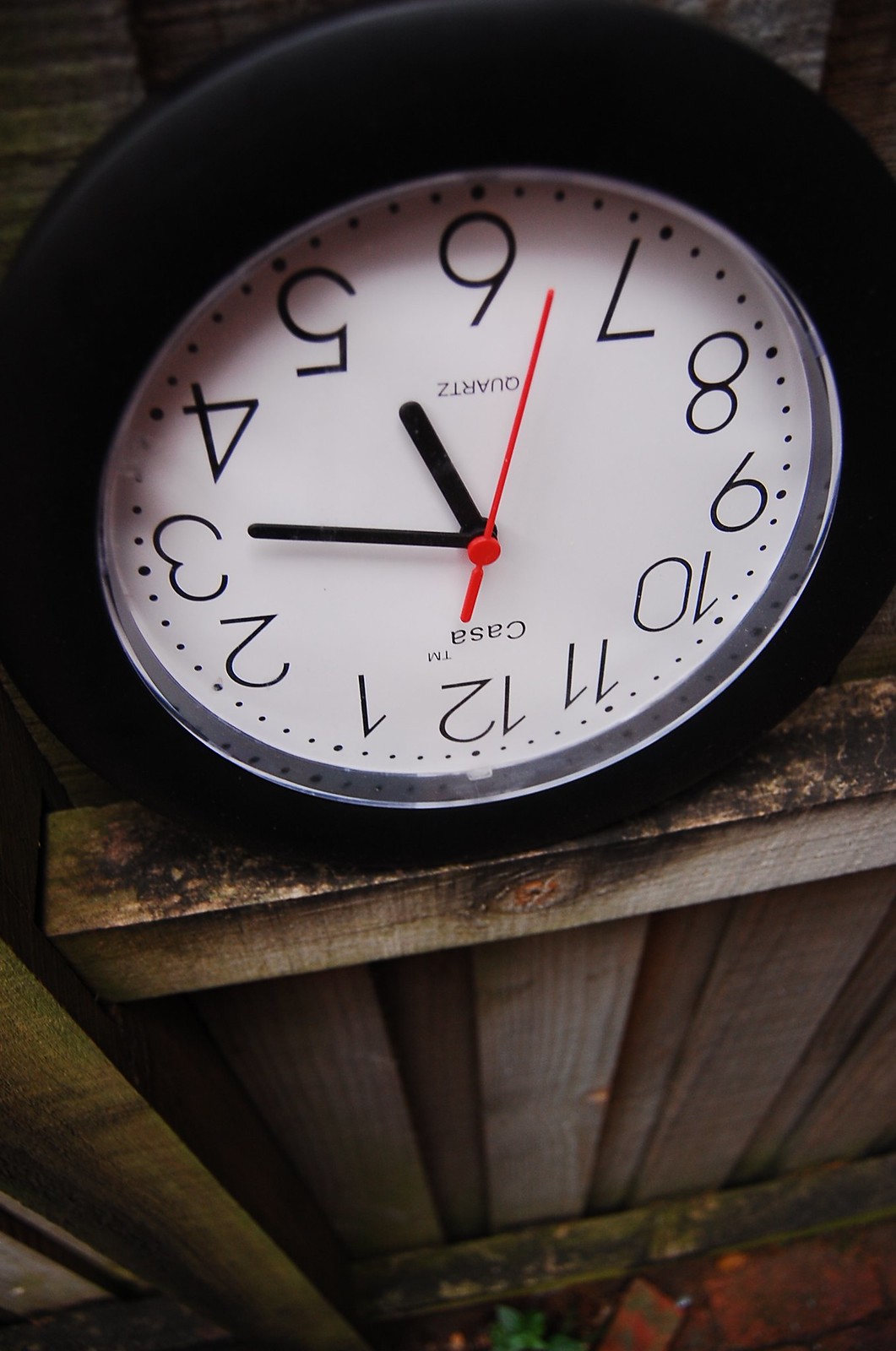The image features a white, round-faced wall clock prominently displaying the brand name "CASA" at the top and "quartz" at the bottom. Although the clock is turned upside down, the time appears to read approximately 5:16. The clock has a black plastic border and black hour and minute hands, with a striking red second hand for clear visibility. It is resting on the ledge of an old, weathered wooden fence, evidenced by the dark discoloration on the wood, giving a rustic contrast to the basic design of the clock.